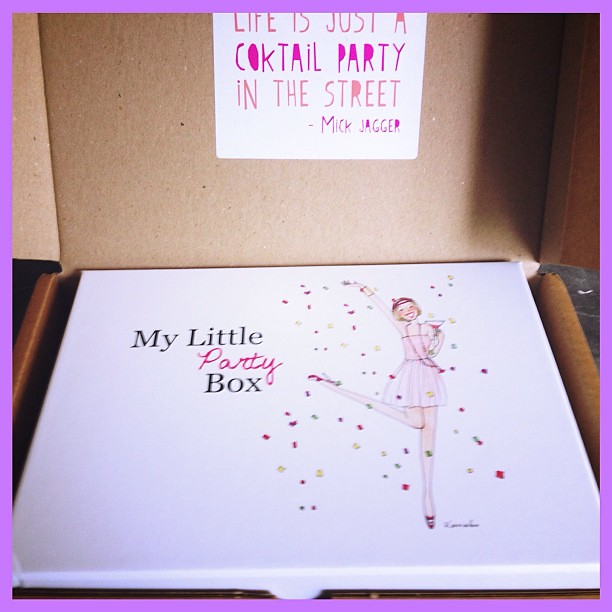The photograph showcases a white box inside a larger brown cardboard box. The lid of the brown cardboard box features a white sticker that reads, "Life is just a cocktail party in the street" – a quote from Mick Jagger, written in vibrant pink and orange colors. The white box inside is labeled "My Little Party Box" in black and pink font. On this box, there's an illustration of a festive blonde woman with short hair, wearing a pink, sleeveless dress that resembles a ballerina outfit. She is beaming with a big smile, her left hand holding a cocktail, and her right leg is playfully lifted in the air. The woman is surrounded by colorful glitter and confetti in shades of red, yellow, and blue. The overall composition is framed by a bright pink outline, adding to the cheerful and celebratory theme of the image.